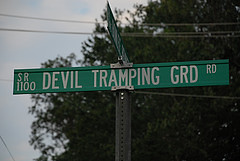The image depicts a very small, color photograph taken outdoors in a landscape orientation, focusing on a typical North American street sign held up by a vertical, circular black pole. The street sign, green with white writing, features "SR 1100" on the left and the vertically stretched name "Devil Tramping Ground Road" in the middle, with "RD" in the top right corner. Behind the sign, underexposed dark green foliage of a large deciduous tree is visible, casting a slight shadow. Telegraph or electric wires stretch horizontally across the top of the frame, slightly sagging. The background sky is mostly filled with white clouds, with a few patches of blue sky peeking through. An intersecting street sign, positioned perpendicularly, is also present but unreadable from this angle. The photograph captures the scene from a low angle, giving the impression of looking up at the road sign on an overcast yet not gloomy day.